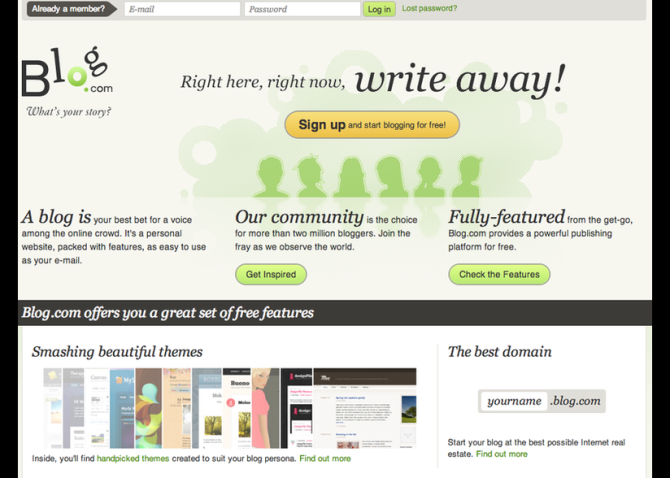This image captures the sign-up and login page for Blog.com, a popular blogging platform. In the top-left corner, the Blog.com logo is prominently displayed, accompanied by the tagline "What's your story?". The main headline on the page cleverly reads "Right here, right now, write away," playing on the word "write" to emphasize the instant gratification of starting a blog. Below this headline, there is a prominent button inviting users to sign up and start blogging for free.

The page is inviting both to returning users, offering a straightforward sign-in process, and to newcomers, providing information on how to sign up and start their own blog. Additional features highlighted on the page include access to various blog themes and the ability to create a custom domain name, formatted as yourname.blog.com. The site likely hosts thousands of blogs and bloggers, fostering a vibrant and diverse community. Users can either sign up immediately or scroll down to further explore the features and benefits of Blog.com.